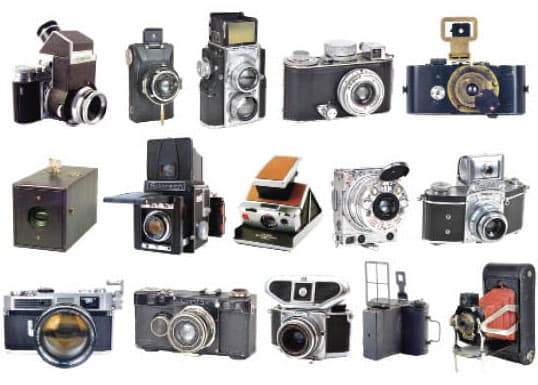The image showcases a pristine white background featuring three rows of vintage cameras, with each row containing five different cameras, making a total of fifteen. The cameras vary in shapes, sizes, and historical periods, with the majority being handheld film cameras, indicating their age and pre-digital era design. In the bottom right corner, there is a distinctive, very old camera featuring an accordion-style extending lens, highlighting its early 1900s origin. Noteworthy cameras include a top-left model with a circular viewfinder on the top, resembling an old box camera, and a mid-row center camera identifiable as a Polaroid, suggesting immediate film production capability. The predominant colors of the cameras are black, gray, and silver, with a few featuring colored panels, providing a glimpse into their varied designs and functionalities.